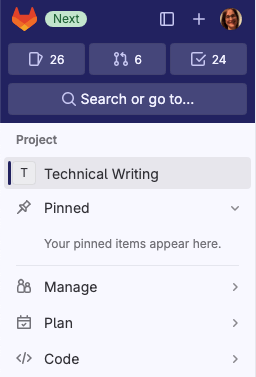This image appears to be a cropped screenshot taken from a phone browser, limiting the visible details about the phone model. In the top left corner, the app's icon, characterized by an orange, minimalistic geometric shape resembling a fox head with two spikes as ears, is noticeable. Adjacent to this icon is a green button labeled "Next." The top section also features a clickable rectangle, a plus icon, and a profile photo of a woman with long hair.

Below this upper segment, there are three icons in sequence:

1. A rectangle icon with the number 26 next to it.
2. An icon depicting a couple of circles connected by a line or an arrow, marked with the number 6.
3. A square icon with a checkmark inside, accompanied by the number 24.

Below these icons, a search icon allows users to search or navigate, indicated by the line "search or go to..." and followed by "..."

Further down, the screen lists sections titled "Project" and "Technical Writing." Under "Technical Writing," there are four subsections: "Pinned," "Manage," "Plan," and "Code." Each subsection title is aligned with a clickable arrow on the right side of the screen. The "Pinned" section is expanded, showing the message "Your pinned items appear here," signifying no items are currently pinned. 

This detailed layout encapsulates the functionality and structure visible in the screenshot.